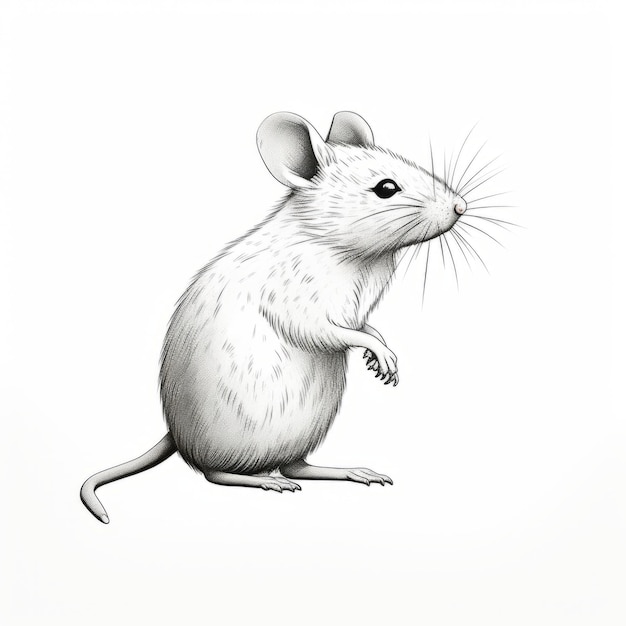This detailed black and white pencil sketch depicts an adorable field mouse centered against a pure white background. The naturalistic and realistic style of the drawing captures the mouse standing upright on its elongated hind legs, facing to the right side of the page. It exhibits a soft, fluffy fur texture interspersed with some darker hairs, and its larger circular ears, almond-shaped dark eyes, and button-like nose add to its cute appearance. The mouse's whiskers radiate in a starburst pattern from the front of its face, and its delicate paws are extended out in front, slightly clenched. The tail curls gracefully into the corner, contributing to the mouse’s distinct and charming look. The image is detailed solely in black, white, and shades of gray, lending it a monochromatic yet lifelike quality reminiscent of a real mouse.